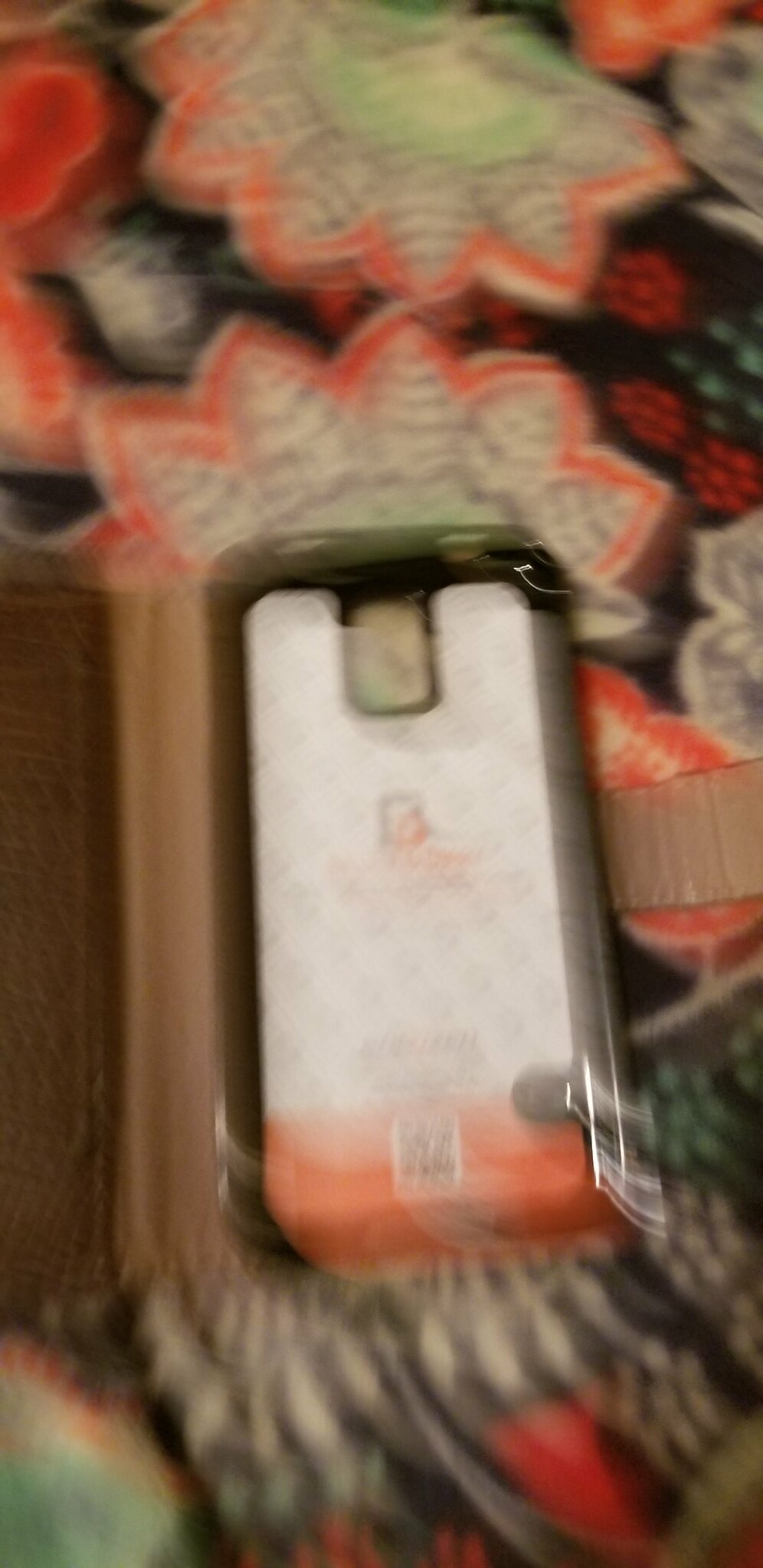This extremely blurry color photograph captures a smartphone placed vertically and face down within a somewhat ambiguous rectangular object, possibly a protective case resembling a book with a leather-like cover. The back of the phone displays a QR code and a central camera lens. Beneath the phone is a distinct, floral-patterned tablecloth, decorated with colorful flowers that include hints of orange, white, red, and green accents, suggestive of a cozy, homey setting. The carpet or tablecloth underneath adds a textured, intricate layer to the scene with its vibrant design.